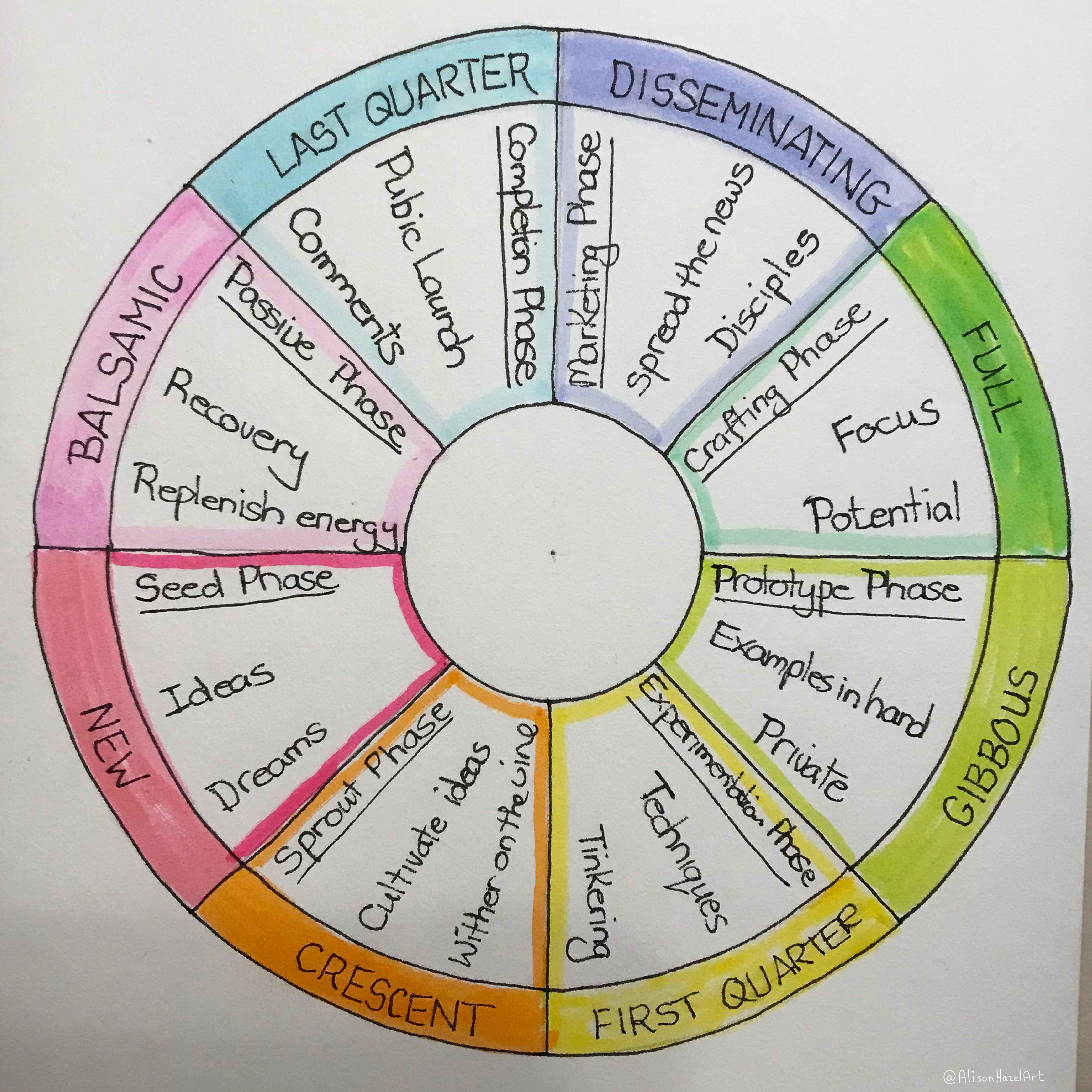The image is a meticulously detailed, square-shaped photograph (5 inches by 5 inches) showing a pie chart drawn on a white piece of paper. This pie chart is effectively a circular diagram, reminiscent of a wagon wheel, divided into eight equal segments, each uniquely colored and labeled. Starting from the top left, the segments change color in a clockwise direction: light blue, purple, neon green, light green, yellow, orange, pink, and a lighter pink.

Each colored segment is labeled with black print, detailing different phases of a process. The light blue segment at the top left is labeled "Last Quarter" and denotes the "Completion Phase," mentioning "Public Launch, Comments." The adjacent purple segment, tagged "Disseminating," is associated with the "Marketing Phase,” highlighting "Spread the News, Disciples." Moving to the right, the green segment is for the "Full" phase, related to "Crafting," with notes on "Focus and Potential," followed by the light green segment marked "Gibbous," which stands for the "Prototype Phase," including mentions of "Examples in Hand, Private."

Continuing clockwise, the yellow segment titled "First Quarter" refers to the "Experimental Phase," emphasizing "Techniques and Tinkering." The following orange segment, labeled "Crescent," signifies the "Sprout Phase," outlining "Cultivate Ideas, Wither on the Vine." The pink segment is marked "New" and corresponds to the "Seed Phase," involving "Ideas and Dreams," and finally, the lighter pink segment at the far left, designated "Balsamic," relates to the "Passive Phase," indicating "Recovery and Replenish."

The segments lead towards and connect to a smaller circle centered within the larger circle, effectively unifying the pie chart and creating a holistic visual representation of the phases. The background of the image shows part of a table in off-white color, adding depth to the photograph.